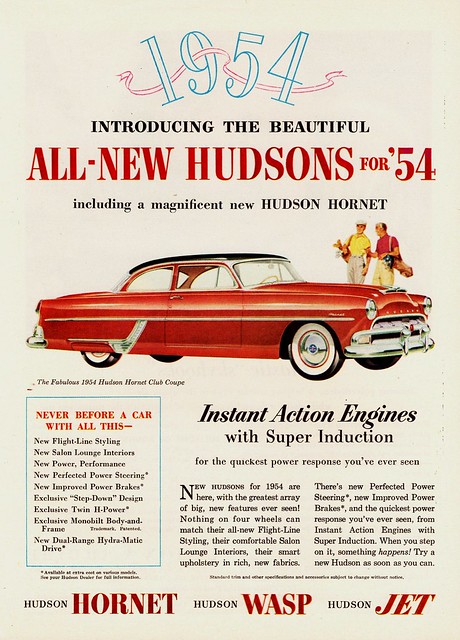This is an advertisement poster from 1954 featuring a detailed drawing of a red vintage Hudson car, specifically spotlighting the all-new Hudson Hornet. The central image shows the car facing right, flanked by two men in the background—one wearing a yellow polo and beige pants, and the other in a red polo and matching beige pants. Both men are carrying golf bags, indicative of a leisurely lifestyle. The backdrop of the poster is light grey, with the main promotional text above and below the illustration. At the top, in blue letters intersected by a red banner, it reads, "1954." Beneath that, the text proclaims, "Introducing the beautiful, all new Hudson’s for ’54, including a magnificent new Hudson Hornet," in black and red typography. Additional text at the bottom lists various Hudson models—Hudson Hornet, Hudson Wasp, and Hudson Jet—alongside detailed descriptions of innovative features such as "instant action engines with super induction," "new flight-line styling," "new salon lounge interiors," "new power performance," "new perfected power steering," "new improved power brakes," "exclusive step-down design," "exclusive twin H power," "exclusive monoblade beauty and frame," and "new dual range hydromatic drive." The image emphasizes the car’s advanced engineering designed for the quickest power response and superior driving experience ever seen. The major colors in the poster are white, black, red, yellow, and various shades of light brown.